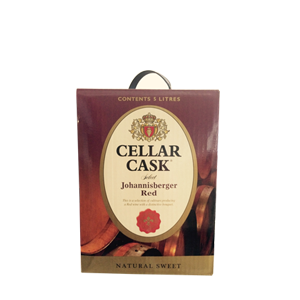The image showcases a box of wine labeled "Cellar Cask Johannesburger Red." The rectangular box features a rich reddish background that becomes lighter towards the bottom. At the top of the box, there is a plastic handle with the text "contents 5 liters" displayed below it. Central to the design is a vertically oriented oval with a beige background and gold trim containing the product name in bold black text. Above "Cellar Cask" is a gold crown emblem with a red crest in the middle. Beneath the text "Johannesburger Red," there is a noticeable red seal. The bottom of the box is accented with a gold band that bears the inscription "Natural Sweet" in black text. In the background, partially visible wooden barrels add a rustic touch to the vignette.